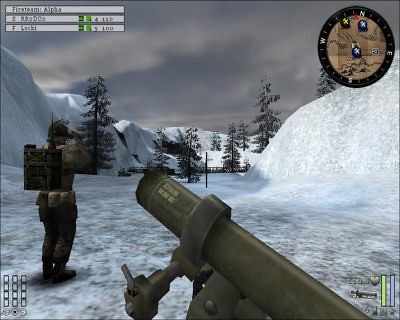In this video game scene, the player finds themselves in a snowy landscape characterized by a flat, snow-covered ground flanked by rocky, snow-laden hills on either side. Scattered pine trees peek from the background, adding to the wintry atmosphere. The focal point is a player dressed in full combat camouflage—camouflage pants, jacket, baseball cap, and sturdy boots—immersed in reconnaissance as he peers through binoculars. A large, brown, and heavy square backpack is strapped to his back, suggesting he's prepared for an extended mission. In the immediate foreground, a machine gun mounted on a stand points ominously at the player, adding tension to the scene. The game's HUD features a round compass in the top right corner, marking the cardinal directions: north, south, west, and east. In the top left corner, three white horizontal bars are visible, with the top bar labeled "Fire Form Alpha," followed by two lines likely representing the players and their scores.